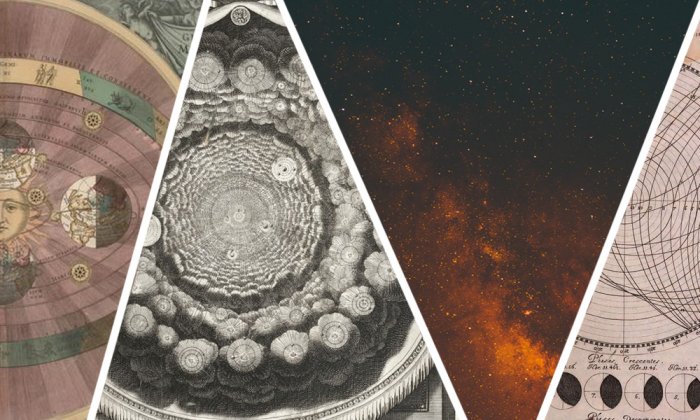The image is a highly stylized and abstract representation of the cosmos, divided into four distinct triangular quadrants, each featuring different celestial themes. The first quadrant, positioned on the far left and pointing downward, is rendered in shades of pale pink, sage green, and beige. It depicts a human face encircled by planets, with angels illustrated in the top left, all centered around a sad-looking sun.

The second quadrant, a black-and-white triangle pointing upward, exhibits gray and white images with circular, concentric patterns resembling the center of a flower or possibly a black hole. This section has a detailed rim and rests on a square background.

The third quadrant, flipped downward and characterized by rust and orange hues, presents a scene of constellations and the night sky. It transitions from dark at the top to bright orange at the bottom, evoking images of stars and a nebula or galaxy.

The fourth and smallest quadrant, an isosceles triangle on the right, features old pen and ink sketches portraying cosmic representations, including four partial eclipses at the bottom. This section is set on a pale beige background with scientific notations and focuses on the phases of the moon or planetary tilts, blending various astronomical and astrological elements.